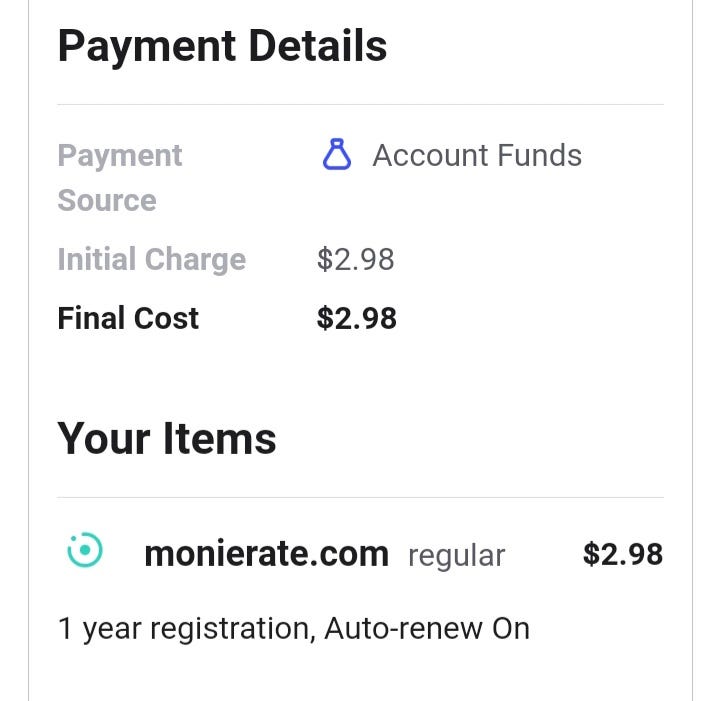This image is a screenshot taken from a web application on a mobile device, featuring a white background and black text. At the top, in large bold black letters, it says "Payment Details." Directly below this title, there is a small gray dividing line. The subsequent section is titled "Payment Source" on the left-hand side, with "Account Funds" displayed to the right. Below this, "Initial Charge" is listed, followed by the amount "$2.98." Beneath that, "Final Costs" is also shown as "$2.98." 

The next section, titled "Your Items" in big bold letters, is separated by another gray divider line. Accompanying this section is a small teal circle featuring an incomplete boundary with a dot in the center. The text "monerate.com" (spelled out as M-O-N-E-R-A-T-E dot com) is displayed, detailing a regular charge of $2.98 for one year of registration. Additionally, it is noted that auto-renewal is turned on.